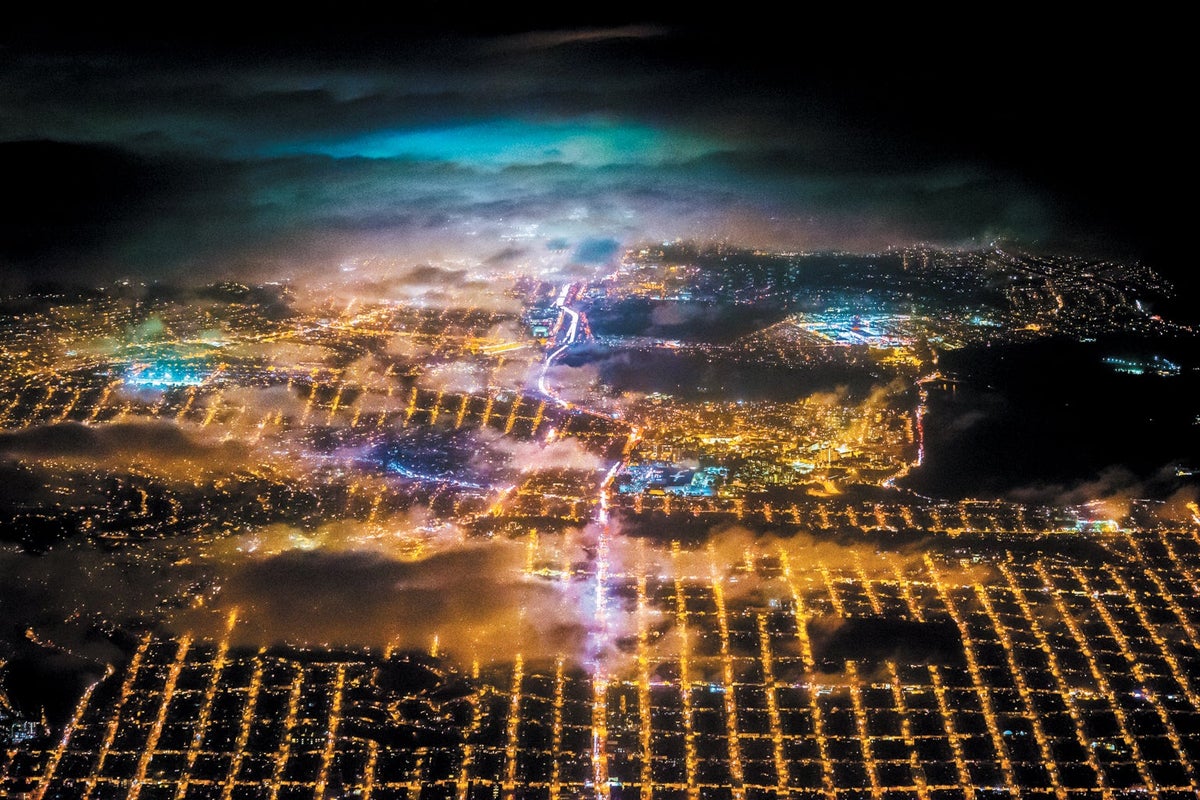The image depicts an aerial view of a city at night, showcasing a meticulously organized grid of bright yellow-orange lights that represent the streets. The scene is accentuated by sections of strikingly vivid colors amidst the primarily orange-lit grid: patches of blue-green, pink, and purple, particularly in the clouds hovering above the city. A prominent main road bisects the image from bottom to top, standing out due to its intense brightness. To the left, clouds obscure parts of the city, adding to the mystical ambiance with their neon green, blue, and pink hues. The far right showcases a more traditional cityscape with illuminated windows, while a significant portion in the middle right appears devoid of lighting. The overall setting is framed by a mix of dark and brightly lit clouds, enhancing the otherworldly feel of the scene.